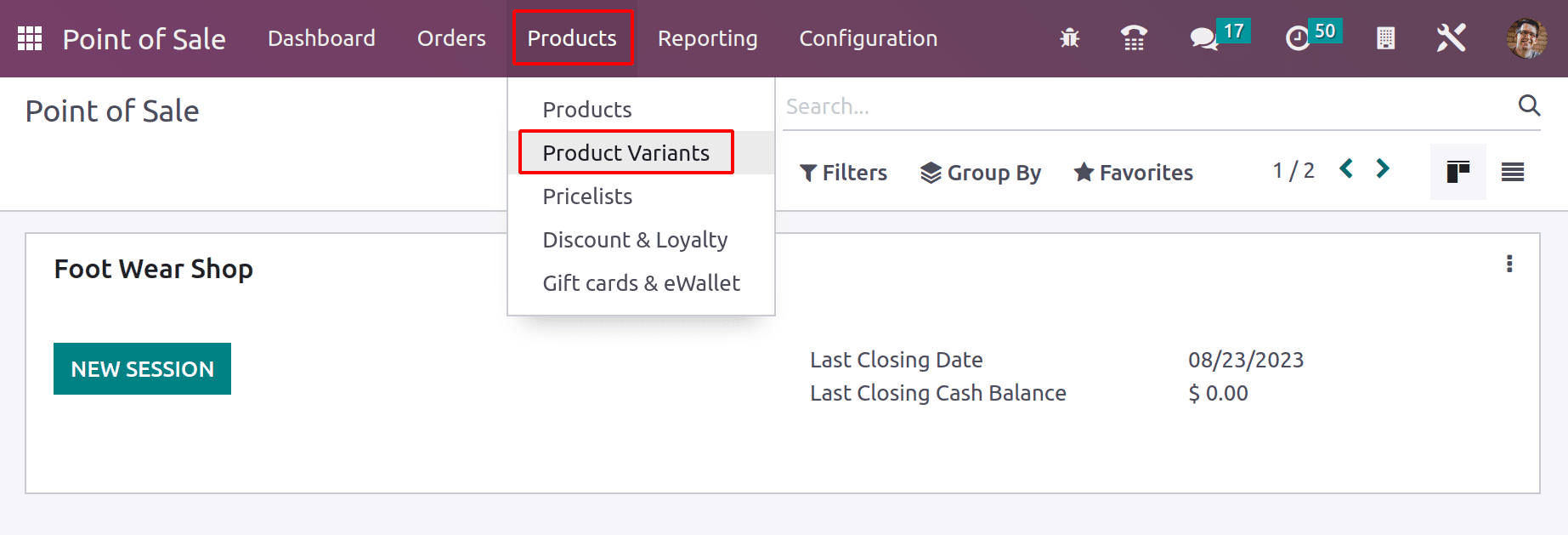In the image, we observe the interface of a Point of Sale (POS) website. At the top left corner, the website's name, "Point of Sale," is displayed. Adjacent to this, there is a logo consisting of a square formed by an arrangement of smaller white circles.

To the right of the logo, a navigation menu features several categories: Dashboard, Orders, Products, Reporting, and Configuration. Further along to the right, there are multiple icons: a bug, a telephone, a chat bubble with the number 17, a clock with the number 50, a note paper, a wrench, and finally, a user's profile picture at the extreme top right.

Beneath the "Products" category, there is a submenu listing options such as Products, Product Variants, Price Lists, Discount and Loyalty, Gift Cards, and eWallets.

Towards the bottom middle-left section of the image, the label "Footwear Shop" is displayed with the option "New Session" directly below it. On the far right within this section, it notes "Last Closing Date: 08-23-2023." Below "Last Closing Date," there is a mention of "Last Closing Cash Balance," which is marked as $0.00.